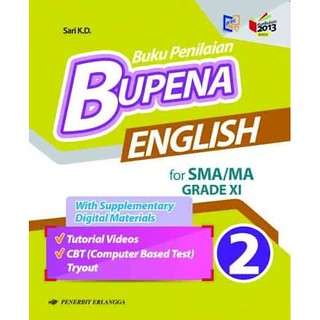This image appears to be the cover of a book titled "Boku Penileiyan Bupena English for SMA-MA Grade 11." The cover features a blend of vibrant colors, predominantly yellow at the top and bottom sections, with additional hues of white, light blue, green, purple, pink, and brown. The central text prominently displays the word "English" on a burnt sienna background, bordered by the same color at the bottom. Emphasizing its educational purpose, the cover mentions supplementary digital materials, which include tutorial videos, a computer-based test (CBT), and a tryout. The background is colorful and dynamic, capturing attention with its multi-colored design. The author's name, "SARI KD," is positioned in the upper left corner, adding a personal touch to the book. The book appears to be rectangular in shape, and there might be small text details that are difficult to read due to the language or size of the image.